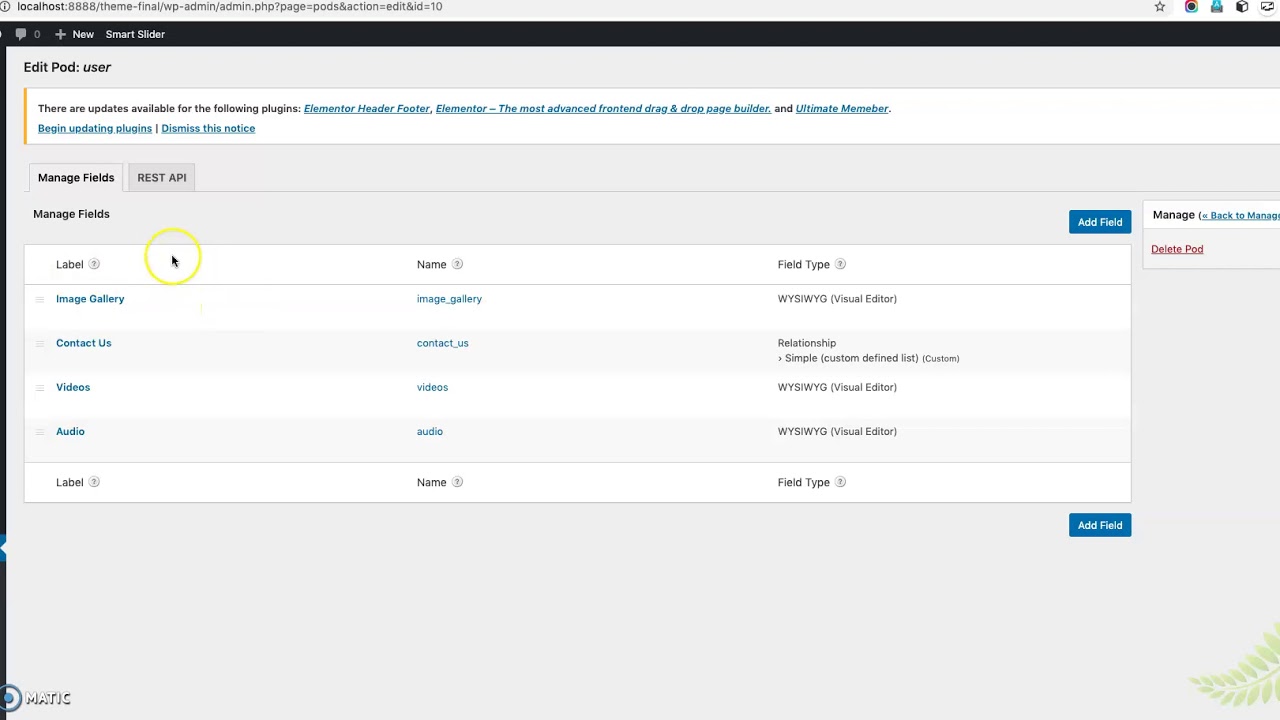The page displayed is a white-themed admin interface for editing a user pod on a localhost server. The interface includes sections for various administrative actions such as managing fields and updating plugins. The header contains elements labeled "Edit Pod User," "localhost," "Theme," "Final Admin," "Admin," "PHP," "Page," "Pods," and "Action."

There is an alert for available updates to several plugins, including Elementor and Ultimate Member. A detailed description under Elementor highlights it as "the most advanced front-end drag-and-drop map builder." Users can initiate updates by selecting "Begin Update Plugins" or choose to "Dismiss this Narrative."

The interface also features a section titled "Manage Fields," boasting an advanced API. Actions available include adding or deleting fields or managing entire pods. A visual indication shows a yellow circle encircling the mouse cursor.

Specific field types available for addition include options such as "Image Gallery," "Visual Editor," "Contact Us," "Relationship," "Videos," and "Audio." Each field type includes an area for a label and name. Lastly, there's a distinct green leaf icon located at the bottom-right corner of the page, adding a subtle visual element to the interface.